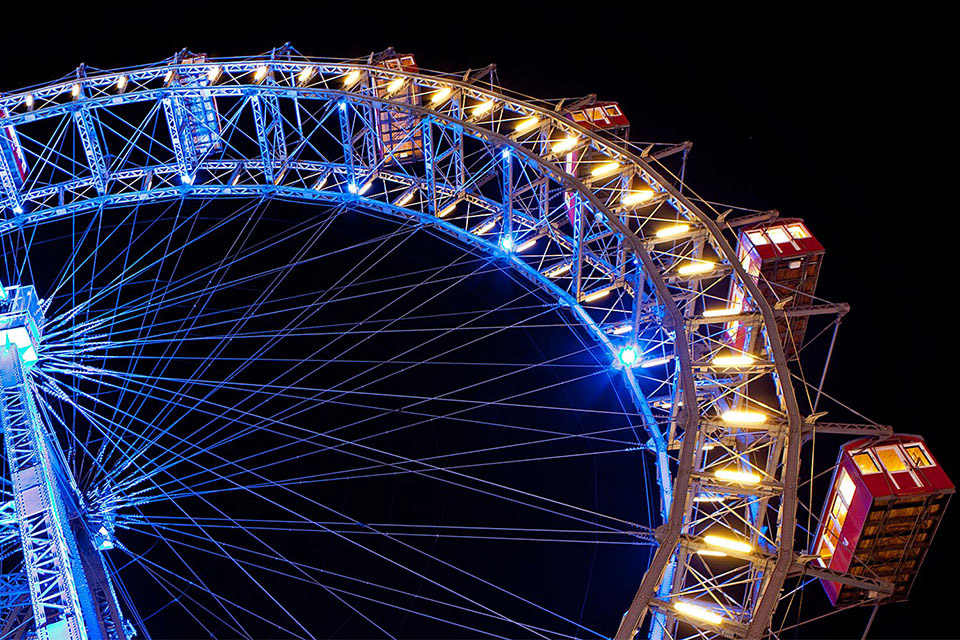This nighttime photograph captures a large Ferris wheel from a ground-up perspective, resulting in an upward view that reveals the intricate details and lighting of the structure. The Ferris wheel is partially visible, with the wheel extending from the bottom left to the upper right of the image. The sky behind is a deep, unfaltering black, devoid of any celestial features, emphasizing the illuminated Ferris wheel.

The wheel is adorned with a vibrant blend of blue lights at its center, transitioning to a warm glow of yellowish-orange lights that highlight the metal spokes and the surrounding structure. This illumination enhances the detailed metal work and showcases the arrangement of horizontal bars and connecting wires.

The passenger cars, which resemble small red train cars or trailers, are fully enclosed with three windows on the front and four on the side. Each car appears capable of holding several passengers, with an estimated capacity of up to twelve people. These cars are evenly spaced around the wheel, and their illuminated interiors contribute to the overall warm, inviting ambiance. The unique perspective and intricate lighting create an impressive and detailed portrayal of the Ferris wheel against the stark backdrop of the night sky.